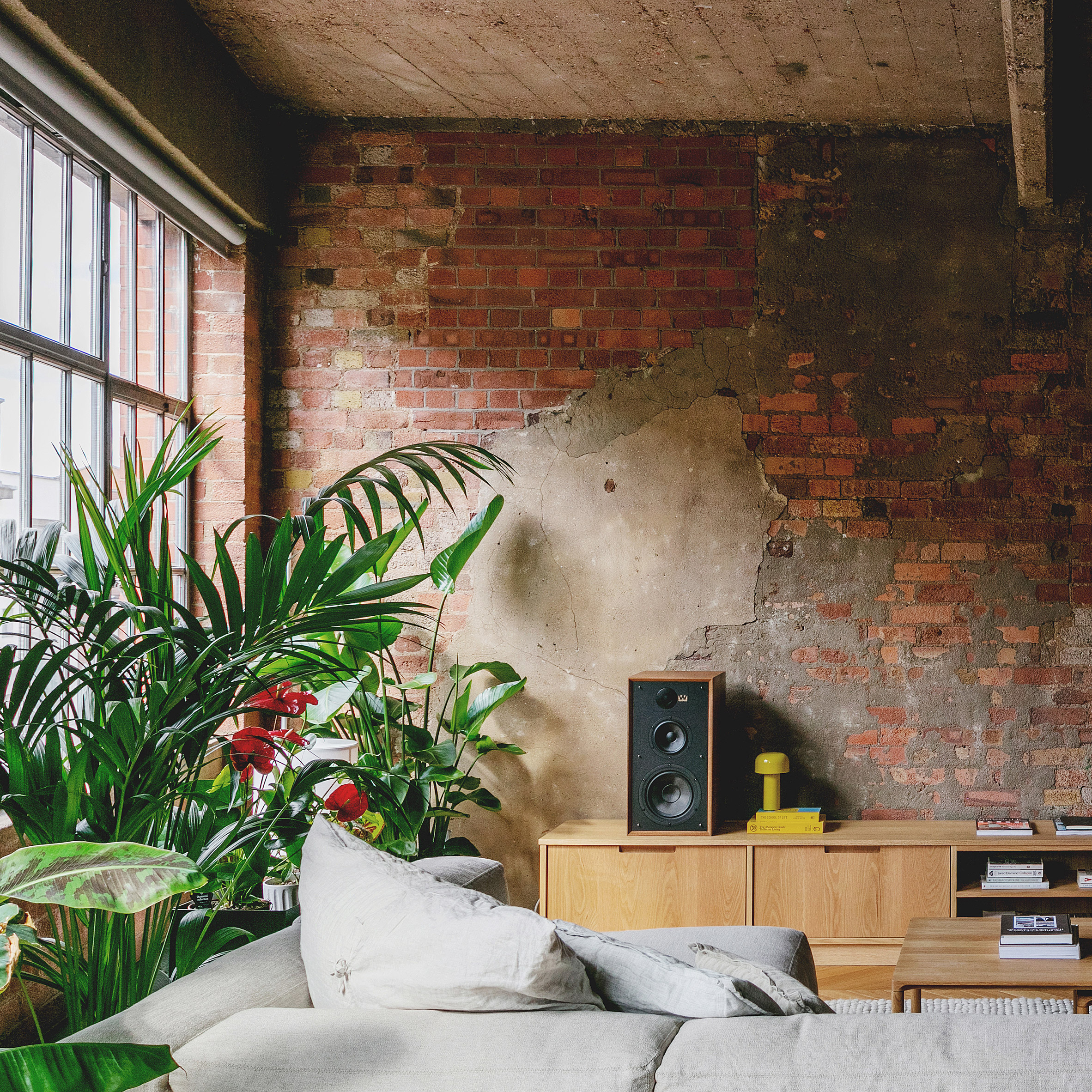This detailed living room exudes a modern industrial charm with touches of rustic warmth. Dominating the space is a large, exposed red brick wall behind the seating area, with areas of cracking and peeling that add character. A distinctive hand-painted profile of a man with a hat in white paint stands out on the brick wall. The room features wooden ceiling beams which complement the brick aesthetic.

In the center, there's a plush couch with white pillows and a textured surface. In front of the couch is a brown wooden coffee table with a glass top, displaying a few stacked books. Partially on a beige rug, the table sits atop a cream rug that adds softness to the setting. To the left of the couch, or slightly forward, stands a black speaker on a sleek metal stand.

A metal entertainment stand, adorned with various books and a yellow mushroom decoration, provides additional storage and style, while tall potted plants with large, light green leaves — likely live plants — offer a natural touch. A profusion of greenery, including long ferns and red-flowered spider plants, graces the room, especially near a large square window with a roll-up shade, contributing to the room's lively ambiance. The variety of plants behind the couch and around the window frames accentuates the room’s inviting atmosphere, merging nature with industrial elements seamlessly.